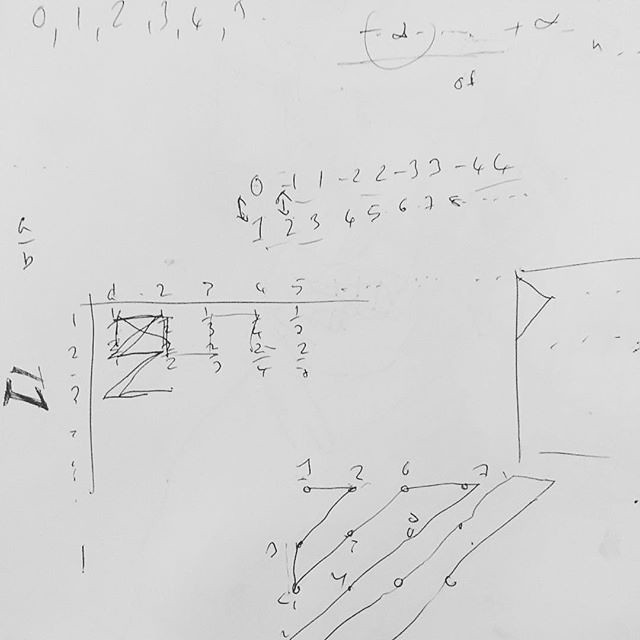A well-worn piece of white scratch paper, filled with a mix of handwriting and various calculations in black pencil, likely used for homework or problem-solving exercises. 

In the upper left corner, the paper features a sequence of numbers: "0, 1, 2, 3, 6" followed by an illegible entry. To the left of this sequence, there's another set of numbers beginning with "-2" and another unreadable part. Below, a line is drawn under the word "of."

Further down, a series of subtractions are listed: "0 - 1, 1 - 2, 2 - 3, 3 - 6, 6." This is followed by another set of numbers: "1, 2, 3, 6, 5, 6, 7, 8."

To the left side, the paper contains the notation "A" followed by a line, and then "B" with "A/B" (A over B). 

On the right side, there is a roughly drawn box, created with either a pencil or pen. Next to this box, another diagram features numbers "1, 2" running down one side and more numerical entries along the top, along with what appear to be fractions mixed in.

Beneath this diagram, additional drawings and calculations with various numbers are visible, though their purpose remains unclear.

The overall impression is a snapshot of a student's process, working through a series of math problems or equations on a plain piece of paper.